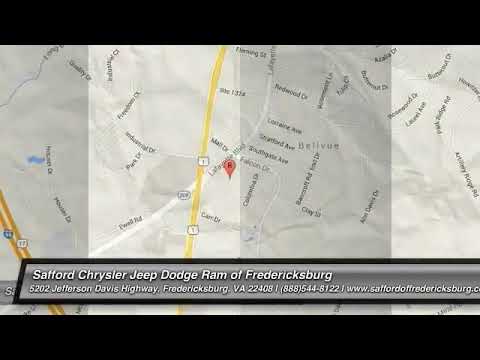The image depicts a digital road map comparable to those found on GPS systems or mapping apps like MapQuest on smartphones. The map prominently highlights "Safford Chrysler Jeep Dodge Ram of Fredericksburg" located at 5202 Jefferson Davis Highway, Fredericksburg, VA 22408. The dealership's contact details, including the phone number 888-544-8122 and the website www.SaffordFredericksburg.com, are displayed at the bottom. The image mainly shows roadways without any topographical features, and includes colors like white, black, yellow, red, gray, silver, and blue. A red pin marks the dealership's location, while yellow lines outline the streets. Despite a six-inch black border framing the top and bottom, the central portion features an intricate map with numerous street names, though many are difficult to read due to the image quality.